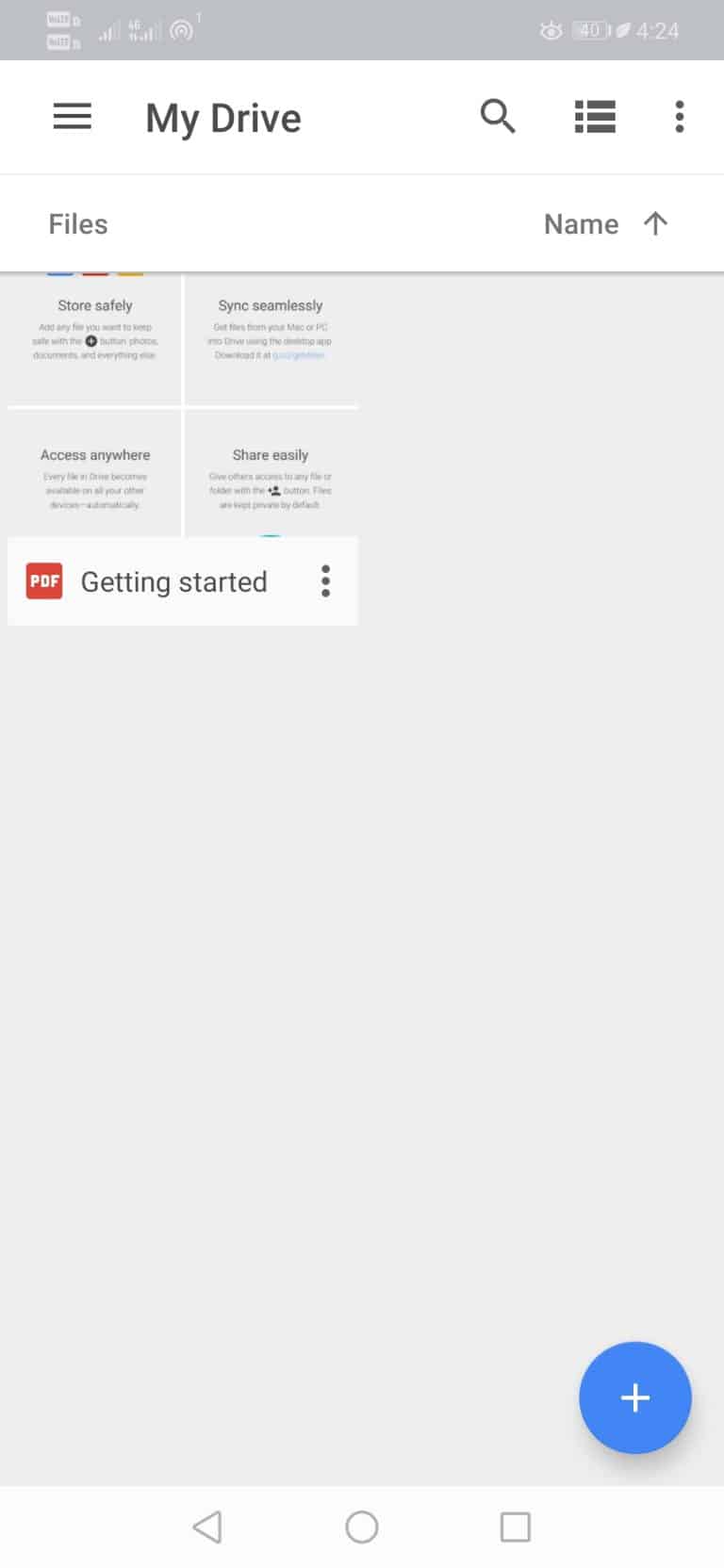This is a screenshot of a Google Drive interface on an Android device, displaying the "My Drive" section at the top in black text against a white background. The screen shows one stored item, titled "Getting Started PDF." A preview of the PDF text reads, "Store safely, sync seamlessly, access anywhere, share easily." In the bottom right corner of the screen, there is a blue circular button featuring a white cross in the center. The bottom of the screenshot includes the standard Android navigation buttons.